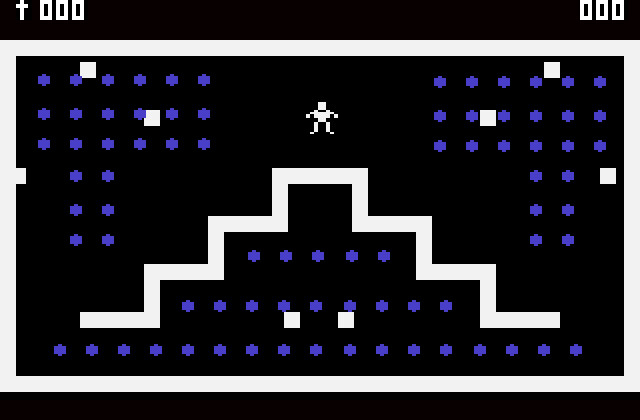This image is a color screen capture of an early video game, possibly for the Atari system, featuring 8-bit graphics typical of the early 1980s. The scene is framed by a white border and set against a solid black background. Dominating the center is a three-tiered, step-pyramid structure filled with purplish-blue dots, symmetrically mirrored from top to bottom. At the pinnacle of this pyramid stands a tiny, pixelated, white silhouette of a person, presumably the player's character. Additional details include two white squares positioned near the bottom of the pyramid. In the upper portion of the image, a black horizontal rectangle serves as the score display. The left side displays a cross symbol followed by three digital zeros, while the right side shows another set of three digital zeros. No text or additional print is present within this minimalist yet intricate scene.